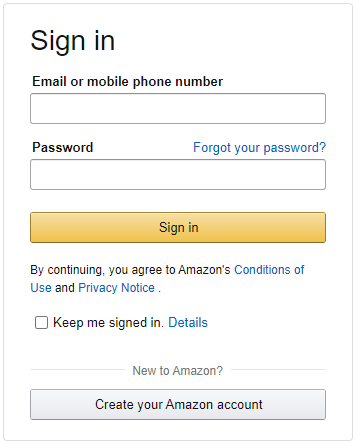The image features an Amazon sign-in page with a clean, structured layout. The page is depicted within a vertically elongated rectangle outlined by a thin gray border on a white background. In the upper left corner, the largest text reads "Sign-In." Below that is a label for "Email or mobile number" accompanied by a horizontally extended input field bordered in gray.

Following this, the page displays the label "Password" with a "Forgot your password?" link in blue on the right side, indicating a path to password recovery. Beneath this, there is another input field similar in design to the one above. Proceeding downwards, a prominent yellow button with black text reads "Sign-In," matching the width of the input fields.

Below the button, there is a declaration stating, "By continuing, you agree to Amazon's Conditions of Use and Privacy Notice," where "Conditions of Use" and "Privacy Notice" are clickable links in blue.

Further down, there is an unchecked square checkbox labeled "Keep me signed in," with an adjacent blue "Details" link.

A horizontal line separates the preceding section from the next, which poses the question, "New to Amazon?" In response, a gray button with a gray outline and black text invites users to "Create your Amazon account." The overall color scheme prominently features black, white, gray, blue, and yellow, ensuring clarity and readability without needing to enlarge the page.